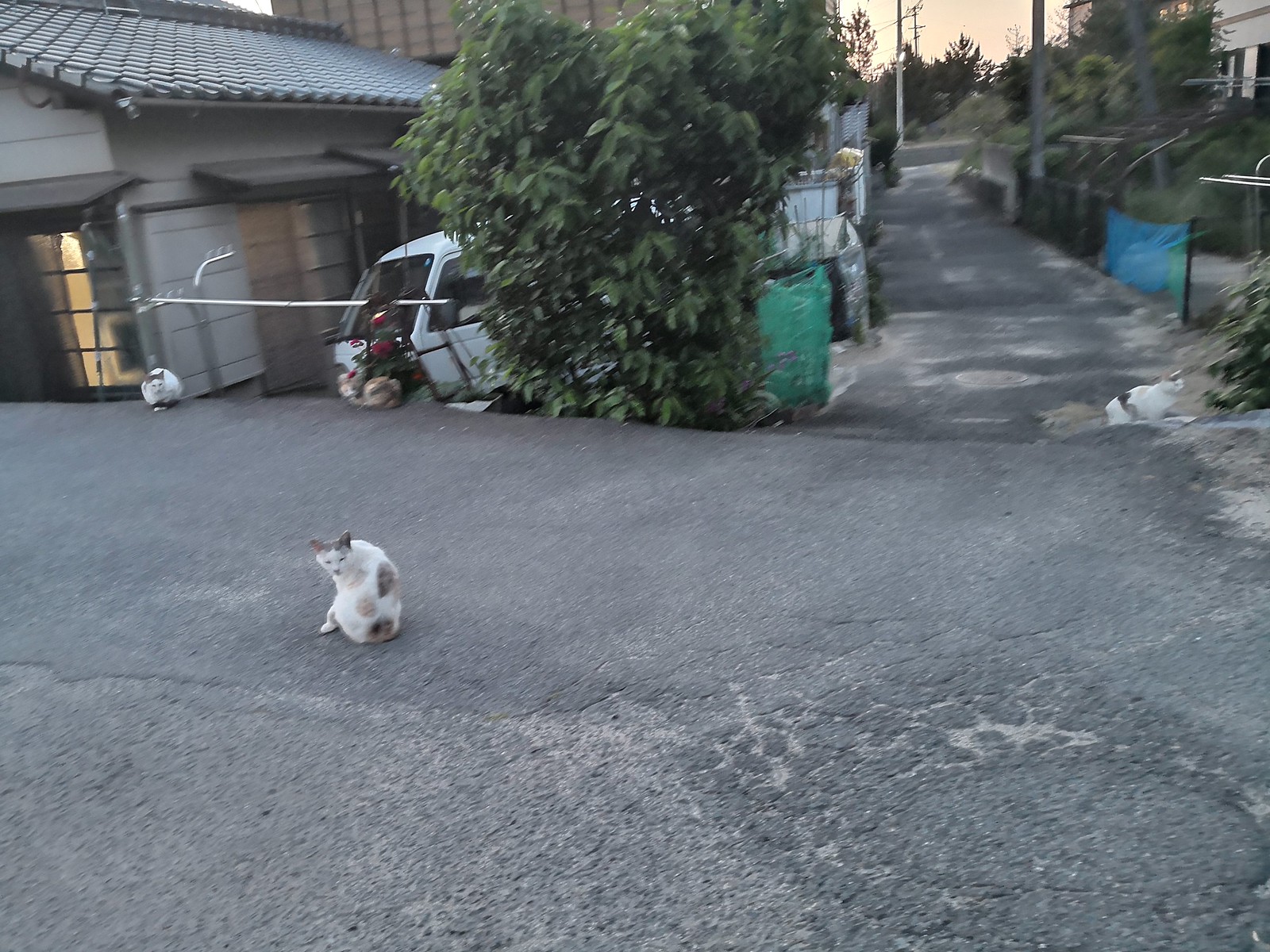This blurry, low-resolution color photo captures a scene in a densely populated, modest neighborhood, likely in Japan. The setting includes uneven concrete pavement and an asphalt street, partially wet from recent rain. The street, aligned with small, single-story homes featuring tan walls and dark brown roofs, extends into an alleyway bordered by puddles. A distinctive step-up area leads to a slightly elevated flat space. Amidst this urban landscape, four cats with short fur and white coats accented by brown and beige spots can be seen: one walking towards the right, two sitting on the street, and another near a green bush beside a typical small white truck parked close to a house. The overall atmosphere suggests either early morning light or late evening dusk.